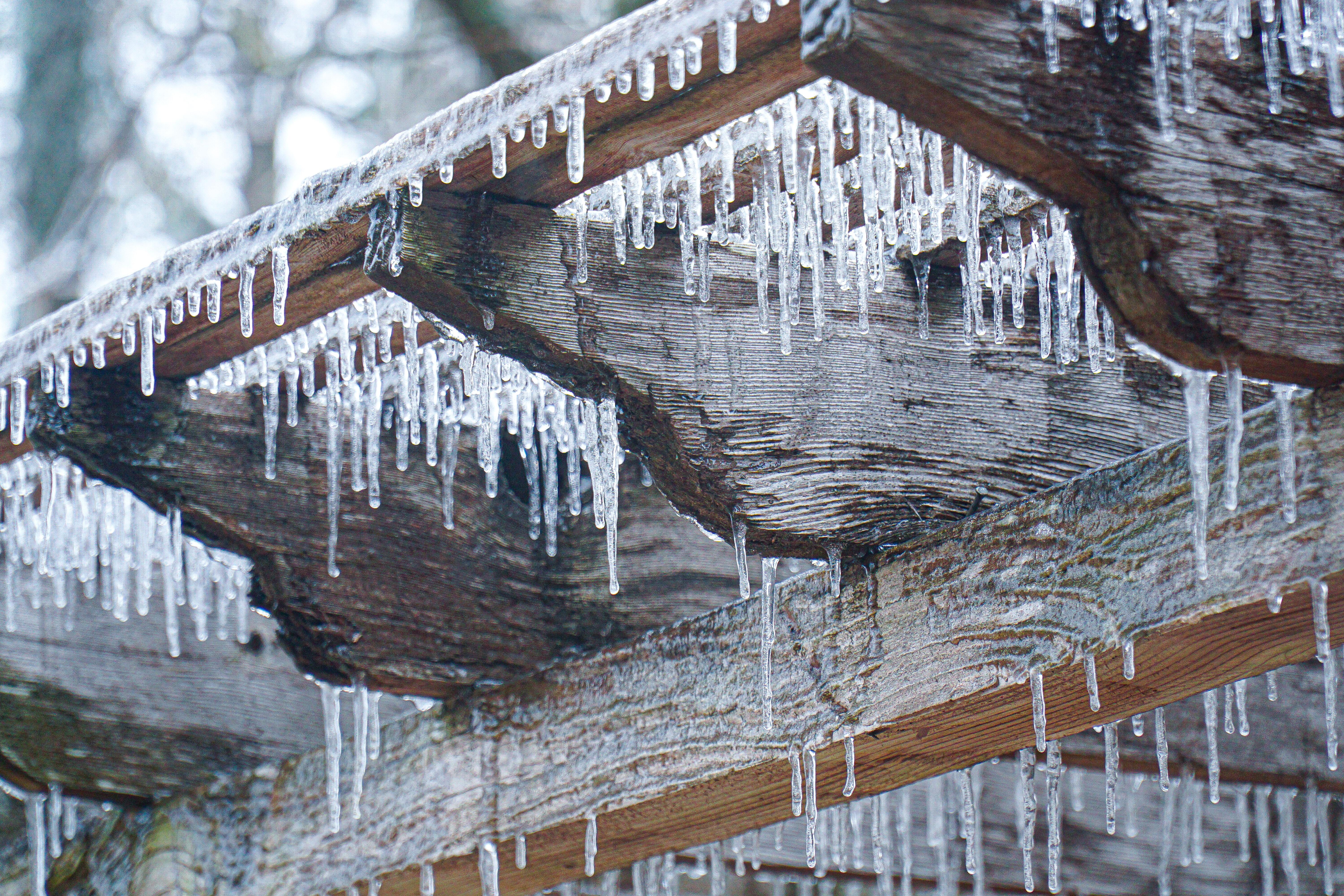This photograph captures a detailed and captivating close-up of a wooden pergola's roof, enveloped in the aftermath of a winter ice storm. The light and dark brown wood beams, with their horizontal streaks, are densely adorned with numerous icicles of varying lengths, ranging from half an inch to about six inches. These icicles create a visually mesmerizing and intricate pattern as they hang uniformly from the wooden structure. The scene hints at the severity of the ice storm, with every surface of the pergola cloaked in ice, implying a thorough freezing. In the background, the bare, leafless trees and the faint glimpse of the sky in the top left corner further emphasize the wintry setting. The overall image is both beautiful and intriguing, showcasing the delicate yet formidable power of nature.